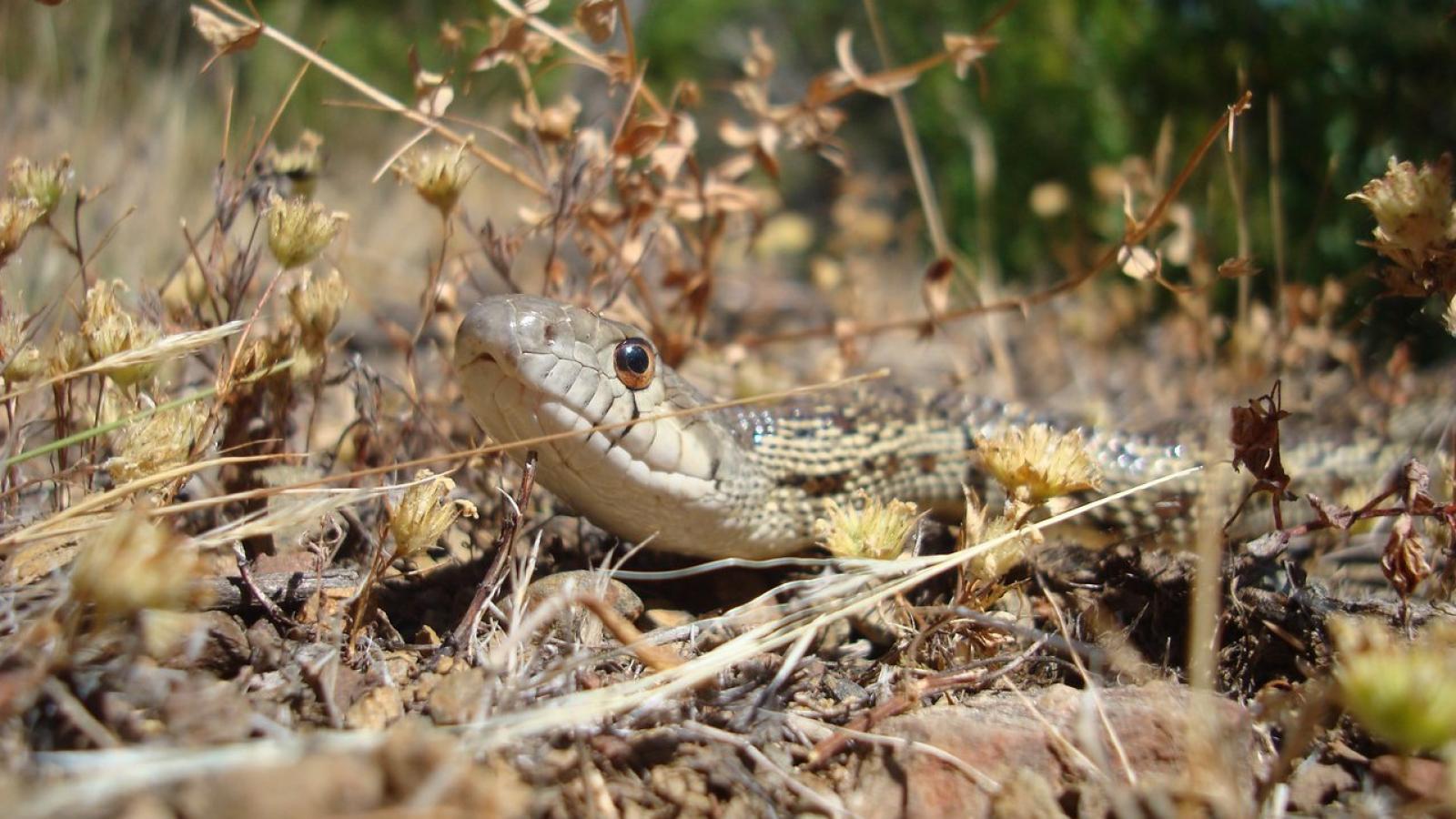In a bright, outdoor, wilderness setting, a light brown snake with darker brown and grayish-white scales slithers across a dirt surface covered in dried, brown leaves, small dehydrated flowers, and dead grasses. The snake’s body is mostly concealed, but its head, tilted slightly upward and adorned with an amber-tinted eye featuring a black pupil, is clearly visible. It blends seamlessly into the earthy background, which includes scattered small rocks and desiccated plant materials, enhancing its camouflage. The background reveals blurry, green trees, suggesting a contrasting, vibrant natural environment beyond the immediate dry area where the snake resides.